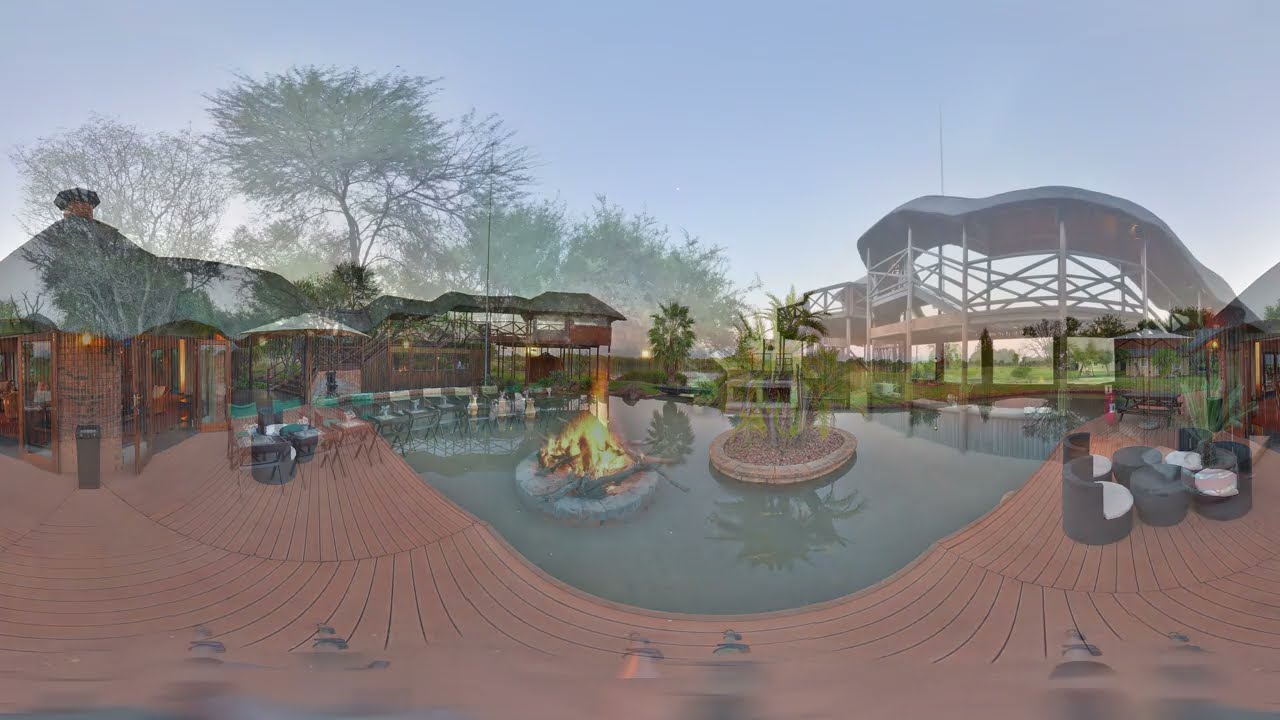The image showcases a serene outdoor resort area centered around a large, well-maintained, oval-shaped swimming pool with brilliantly blue water. Surrounding the pool are various structures including an open patio with wood pillars, providing a shaded lounge area equipped with multiple couches arranged around a square table. Adjacent to the pool, a stone decorative border adds an aesthetic touch, while palm trees and neatly manicured grass enhance the tranquil ambiance. On the left side, a smooth walkway winds through green grass and leads to additional lounges and outdoor seating areas. The scene includes several small sheds or pagodas furnished with sofas and tables, ideal for casual gatherings or dining. Further back are more houses and trees, with paths offering leisurely strolls through this calm, spa-like retreat, devoid of people and inviting in its cleanliness and calm.